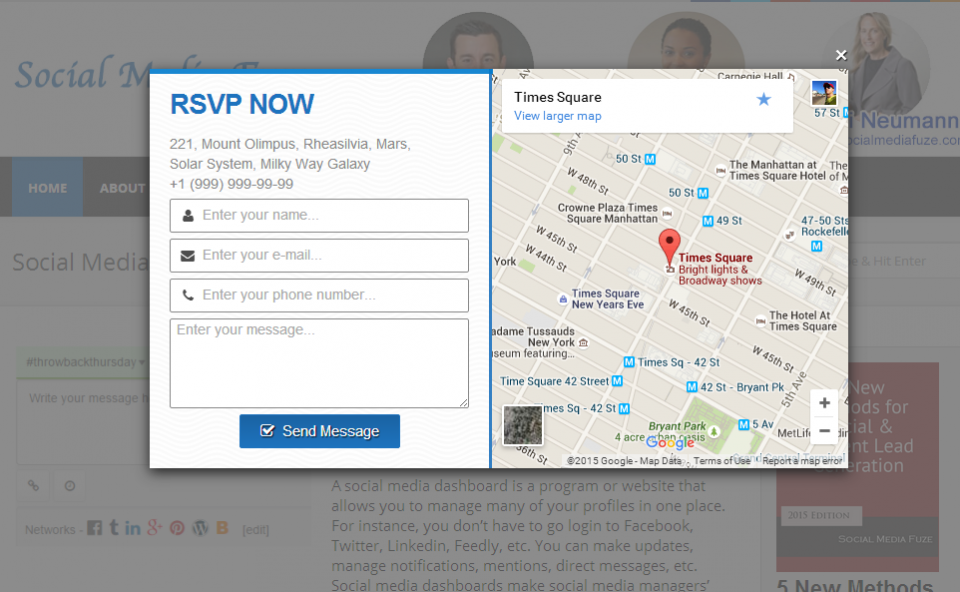A detailed and cleaned-up caption for the described image:

"The image features a greyed-out background with several interactive elements positioned around the frame. On the top left, there is an icon labeled 'Social One.' Adjacent to it, a circular icon contains the image of a woman, accompanied by another woman within the same circle, labeled 'Newman.' Moving left again, there is a 'Home' button, followed by an 'About' section focused on social media functionalities. The central theme of the image appears to be a user interface for a social media dashboard, which is described textually at the bottom.

The highlighted description explains that the social media dashboard is a program or website that enables users to manage multiple social media profiles — such as Facebook, Twitter, LinkedIn, and others — from a single platform. It covers capabilities like posting updates, managing notifications, checking mentions, and monitoring posts.

At the center, the text cryptically references '221, Mount Olympus, Mars, Solar System, Milky Way Galaxy,' followed by a sequence '999-99.' There's also an invitation to 'Enter your email' and 'Enter your phone number' for further engagement options. Additionally, a checkmark signifies completion or verification of a task.

Towards the bottom left, there is a representation of Times Square, marked with larger red map pins linking to notable attractions like bright lights and Broadway shows."